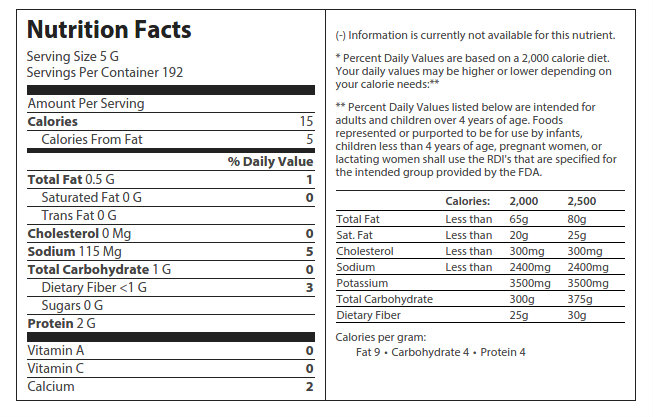The image showcases a detailed Nutrition Facts label for a consumable product on a white background. The label, presented in black text on a white rectangular backdrop, is divided vertically by a thin black line. The left section lists vital nutritional information such as serving size (5 grams), servings per container (192), calories (15), calories from fat (5), and the percentages of daily values based on a 2,000-calorie diet. It breaks down total fat (1%), saturated fat (0%), trans fat (0%), cholesterol (0%), sodium (5%), total carbohydrates (0%), dietary fiber (3%), and protein (2 grams). Additionally, the label includes vitamin A (0%), vitamin C (0%), and calcium (2%). The right section of the label provides further details on daily values and how much fat, cholesterol, sodium, potassium, total carbohydrates, and dietary fiber should be consumed daily on a 2,000 or 2,500-calorie diet. The information also emphasizes how these values contribute to overall nutritional intake.